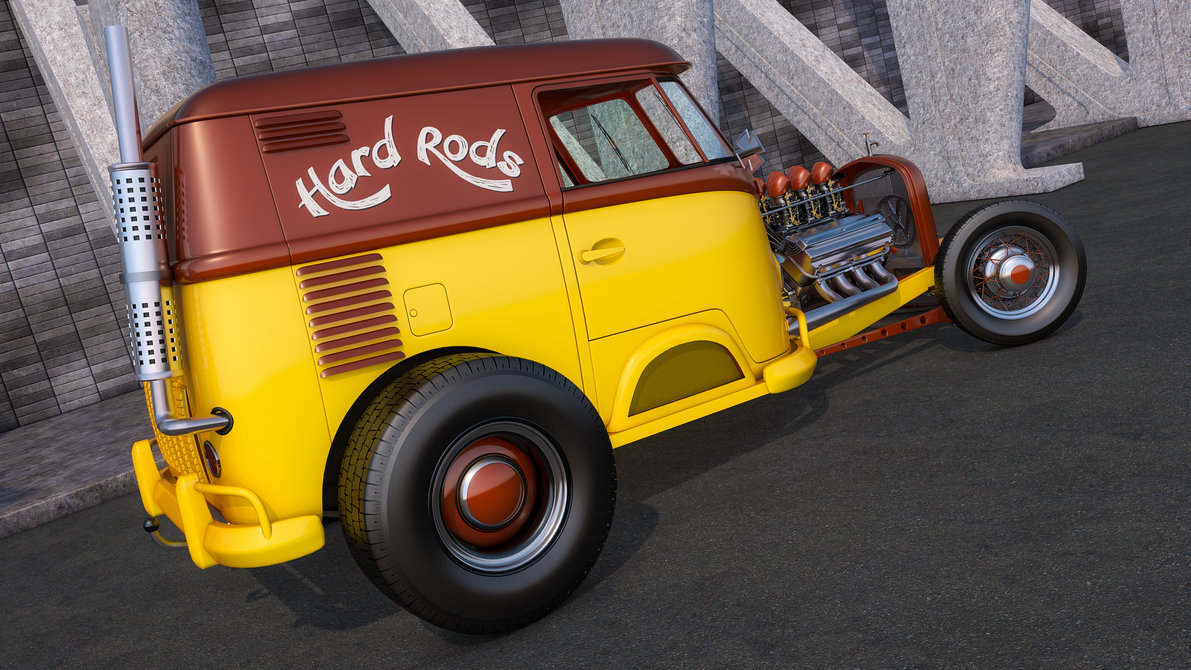The image displays a digitally generated side view of an old-fashioned car with a yellow body and a maroon-brown top. The car's engine is exposed at the front, with no hood covering it, and features a small front wheel and a significantly larger rear wheel. Emblazoned in white letters on the maroon-brown top section, the text "hard rods" is prominently visible. Extending from the rear is a steel muffler tube that points upwards. The car is positioned on a dark gray reflective floor, set against a backdrop of stone gray tiles and light gray columns shaped in a V pattern. The overall scene incorporates shades of gray, with distinctive elements like a gray pavement and a brick-patterned wall adding depth to the setting.